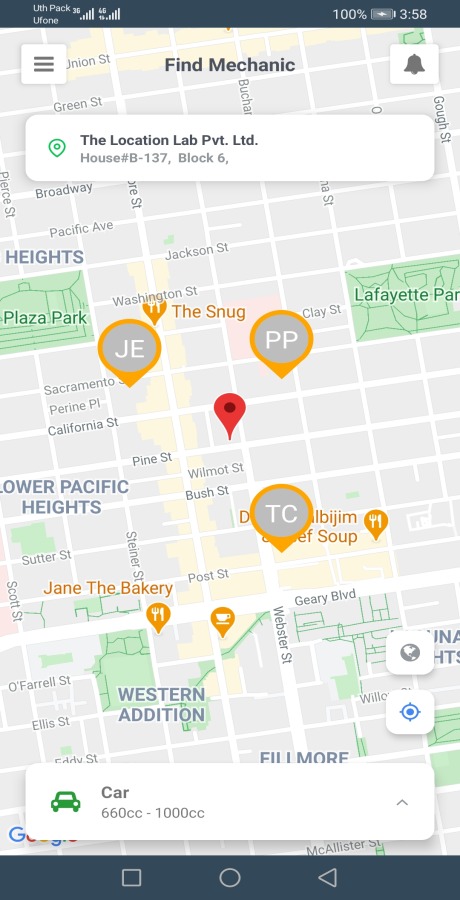The image displays a smartphone screen showcasing a Google Map interface. In the upper-left corner of the screen, the signal strength is visible with the label "UTHPAC UFone." Two sets of cell signal bars are present. On the right side, a battery icon indicates a 100% charge, alongside the number "358." 

Directly beneath this information, the Google Map app is open with the text "Find mechanic location lab PT PVT LTD, house number B-137, block 6." The map highlights several points of interest, including restaurants, marked with pins labeled "JE," "PP," and "TC." However, the exact location of "lab PT PVT LTD" is unclear.

The screen also features a white band at the bottom, containing a pull-up menu labeled "car 660 CC-1000 CC" in gray text. A green car icon is present beside the label. The overall color scheme of the interface includes black, white, gray, green, orange, and yellow elements, with the top part of the screen's text displayed in white font against a black strip background.